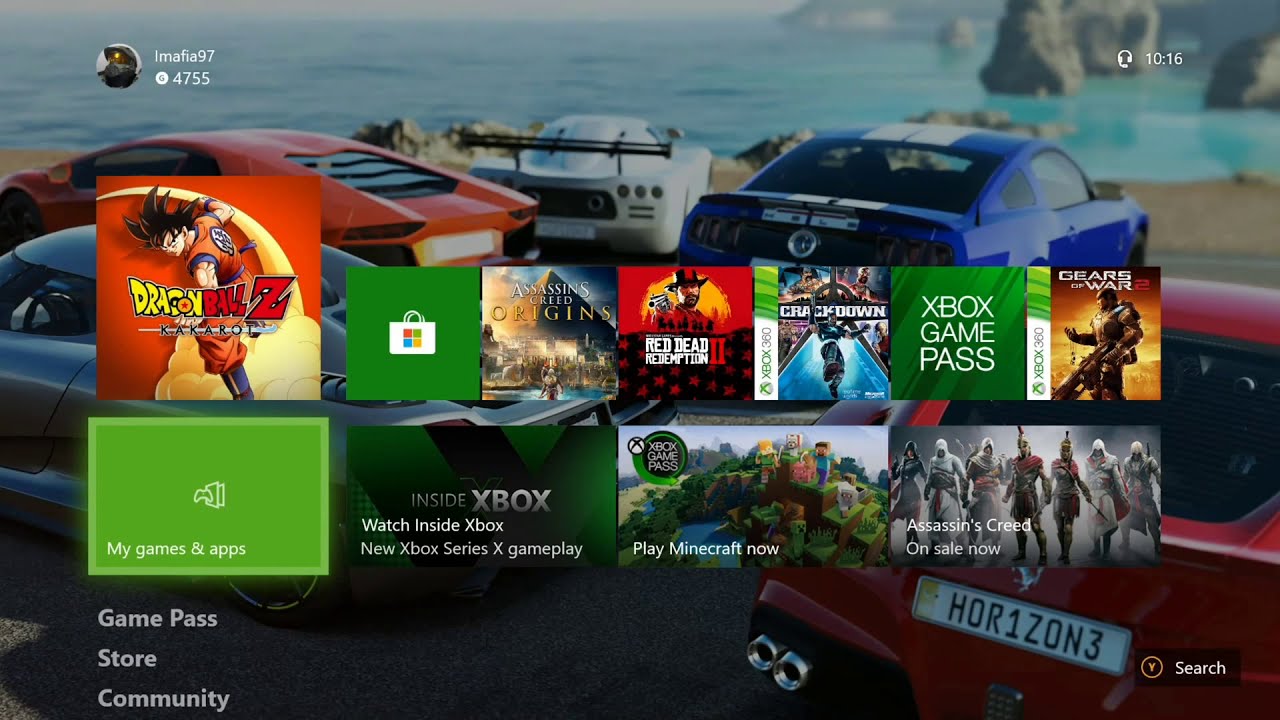This is a detailed screenshot of a computer or laptop monitor displaying a gaming dashboard interface. At the top left corner, there is a circular profile picture followed by the username "El Mafia 97" and a Gamerscore of "4755". To the right of the username, the number "1016" is displayed, possibly referencing points or currency within the gaming platform.

In the background, there are five vividly colored cars—green, red, yellow, white, and dark red—backed up towards one another, arranged in a semicircle. These cars are parked next to a waterway adorned with large rocks, depicted in a stylized video game environment.

Overlaying the background image are various boxes advertising different games and services. The advertisements include titles and features such as:
- "Dragon Ball Z: Kakarot"
- A green box featuring the Microsoft symbol
- "Assassin's Creed Origins"
- "Red Dead Redemption 2"
- "Xbox 360"
- "Crackdown"
- "Xbox Game Pass"
- "Gears of War 2"
- "Inside Xbox: Watch Inside Xbox"
- "New Xbox Series X gameplay"
- "Play Minecraft Now"
- "Assassin's Creed on sale now"
- A green box indicating "My Games and Apps".

The overall display provides a vivid snapshot of a typical gaming experience, highlighting various game options and navigation features within the gaming platform.